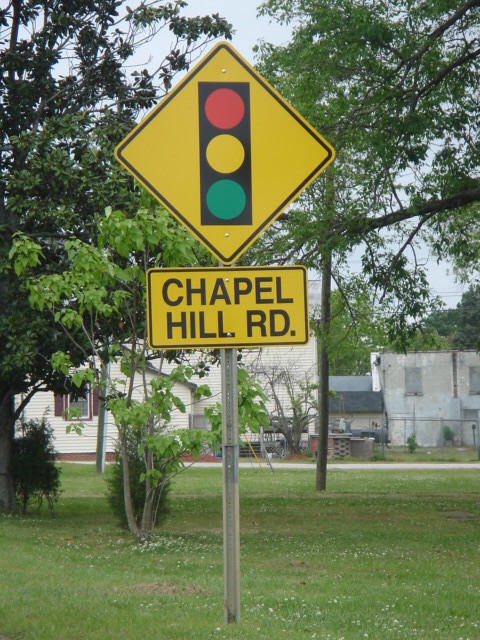The image captures a road scene featuring a yellow diamond-shaped road sign with a clear black outline, indicating an approaching traffic light. The traffic light symbol on the sign displays red, yellow, and green lights aligned vertically. Mounted directly below this traffic sign is a rectangular yellow sign that reads "Chapel Hill Road," both fastened to a single gray post anchored into a grassy area. Surrounding the signs, a few trees and bushes are visible, and in the distance, white portable buildings with windows framed in green and red can be seen. Beyond these, a white house with burgundy shutters and another more dilapidated structure are noticeable. The sky in the background is slightly out of focus, presenting a light blue-gray hue influenced by the weather conditions.